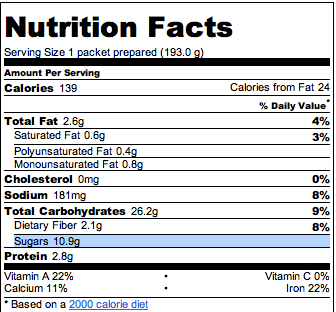This image displays a Nutrition Facts label that appears to be digitally created rather than a photograph of an actual product package. The label itself is white with a thin black border, and the "Nutrition Facts" title is prominently placed in bold, black text aligned at the upper left corner. Below this, the label specifies a serving size of "One Packet Prepared (193.0g)." 

The nutritional information is meticulously organized below a solid horizontal black line, with details about various nutrients. The label indicates that each serving contains 139 calories, including 24 calories from fat. The total fat content is 2.6 grams, which is 4% of the daily value. There is no cholesterol in the product, while the sodium content is 181 milligrams, accounting for 8% of the daily value. The total carbohydrate content is 25.7 grams (9% of the daily value), including 10.9 grams of sugars, which is highlighted with a light blue background. The dietary fiber content is 2.3 grams (8% of the daily value), and the protein content is 2.8 grams.

Additional nutrient information includes iron, which is 22% of the daily value. However, it’s noted that the product contains no vitamin C. Below the nutritional values, blue text indicates that these values are based on a 2,000-calorie diet. The image emphasizes a black-and-white color scheme for the most part, except for the highlighted sugars line and the blue text at the bottom.